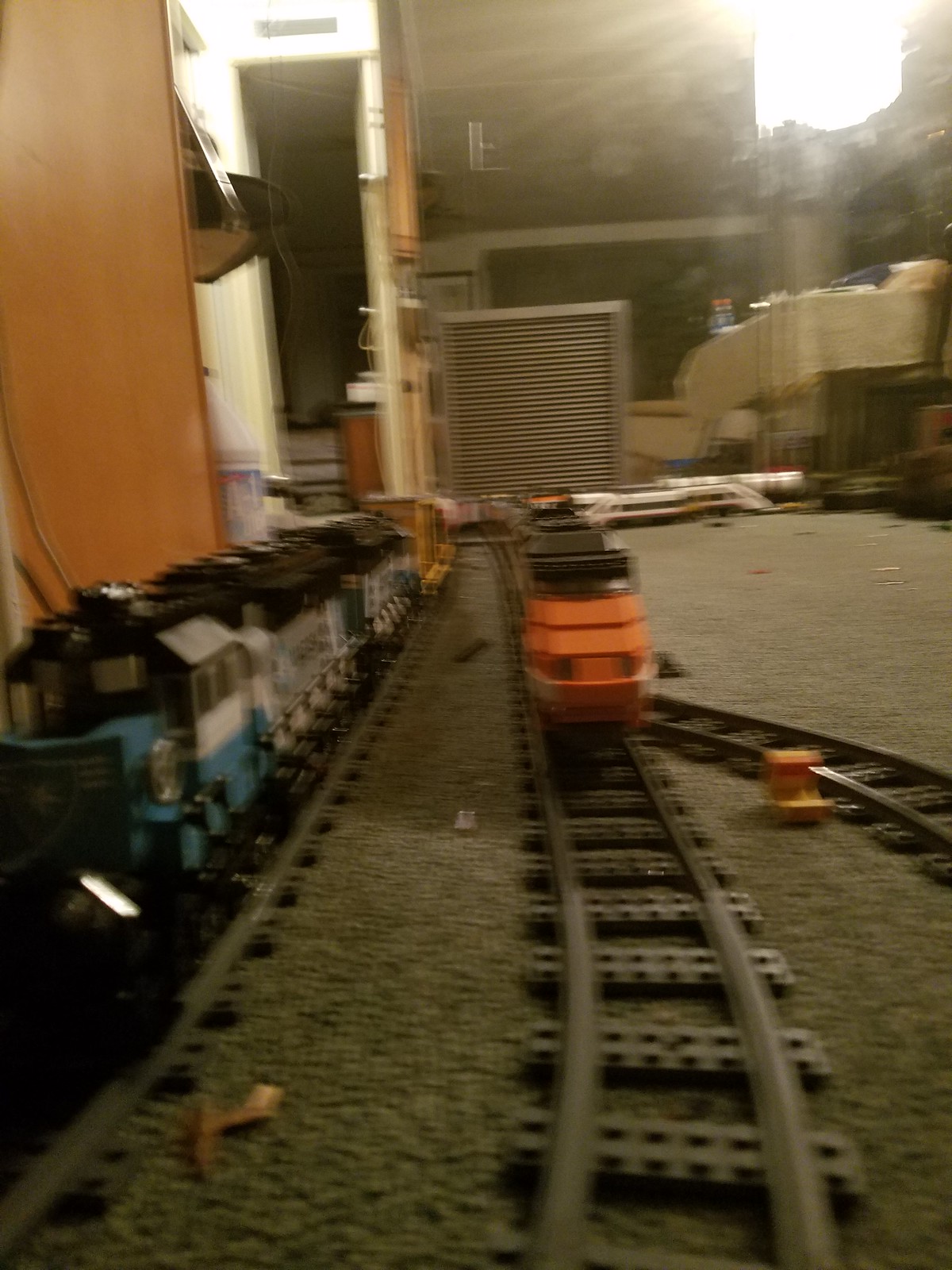The image depicts a scene with toy trains laid out on carpeted tracks in a room. The setup features three converging tracks, creating a complex layout. On the left track, a blue and gray train with a black top is prominently positioned, with several train cars trailing behind, including at least one yellow car, though parts appear blurry. The center track hosts an orange engine with a black top, situated slightly further back and less in focus. Notably, an additional track diverges to the right from this middle track, suggesting a switch for a change in direction. The background reveals various household items, including a TV, a lamp, a wardrobe, cabinets, and possibly a vent, adding to the sense that the picture is taken in a well-lived-in house.